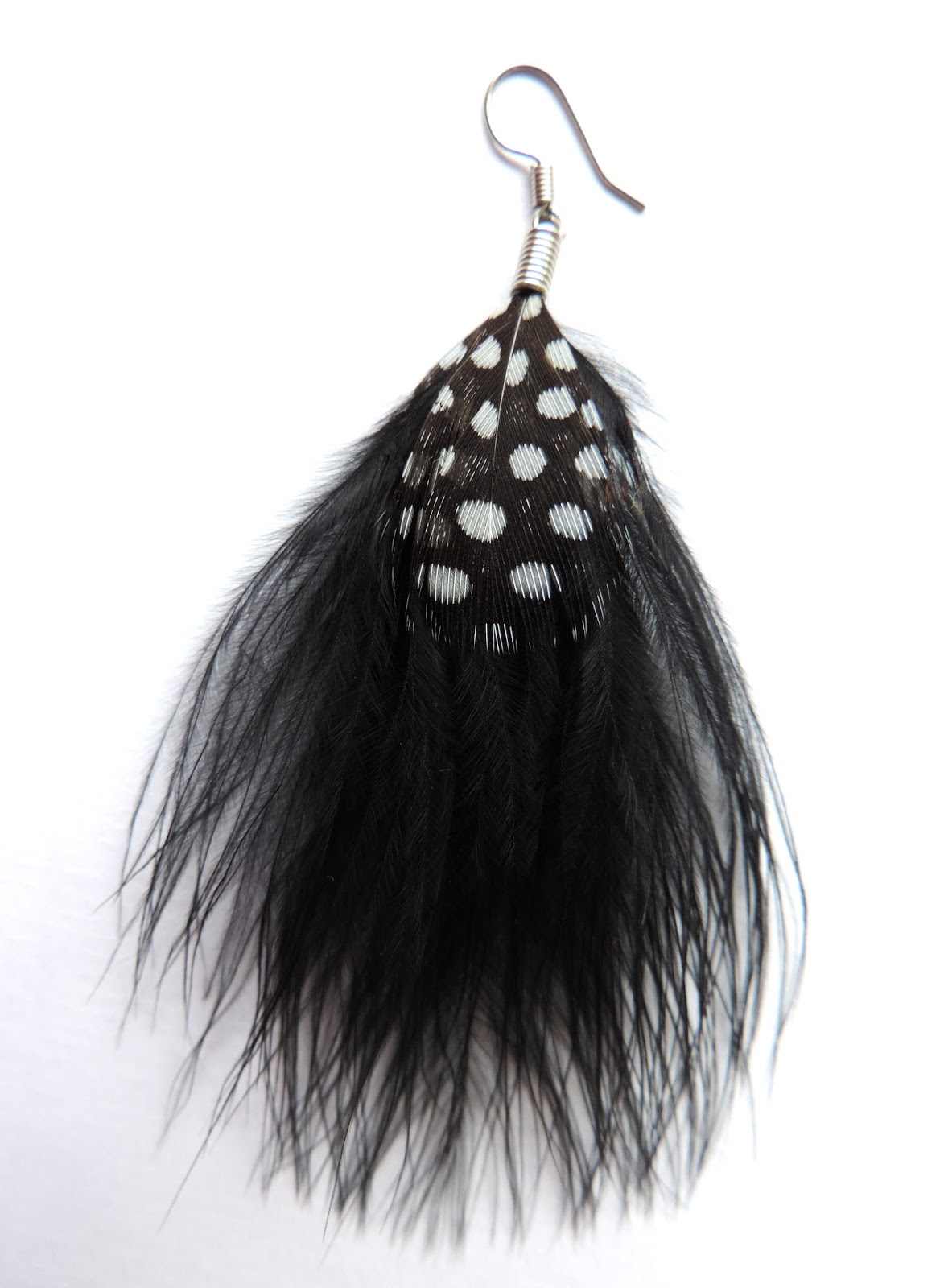A single earring lies on a white surface, prominently showcasing its intricate design. The earring features a silver metallic hook positioned upside down, intended to hang from the ear. Attached to the hook is a striking decorative element composed of thin, black, feathery strands that fan out broadly. These feathery strands resemble the body of a bird, giving the earring a unique and fluffy appearance. Central to the design is a black structure adorned with white polka dots, adding a touch of elegance and contrast. The overall look is both bold and delicate, making the earring a captivating accessory.